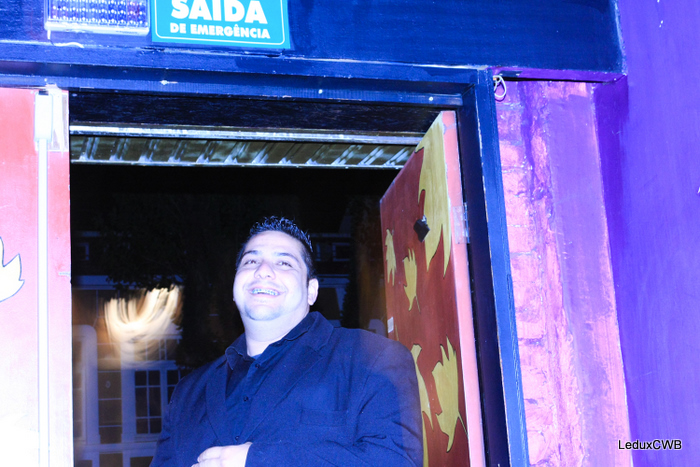The photograph captures a heavyset man standing in a partially open doorway that has been hand-painted in a bright, eclectic mix of colors including blue, yellow, red, pink, and purple. The door itself is predominantly blue, with splashes of other vibrant colors and little leaf designs, giving it a sloppy yet artistic appearance. Above the doorway, a sign is prominently displayed, reading "Saída de Emergência" in light blue against a dark blue background, with a small light fixture illuminating it. The surrounding walls feature irregular purple and pink shades, with a yellow stripe and some sort of design partly visible on the left side. The man in the doorway is around 25 to 26 years old, with black hair and a broad, cheerful smile. He is dressed in a blue suit jacket over a black button-up shirt and his left hand is partially visible. The photograph has a slight blur and in the bottom right-hand corner, the text "Lee Ducks CWB" appears in black. The overall scene gives an impression of vibrant chaos and joy, captured in a moment of candid laughter.